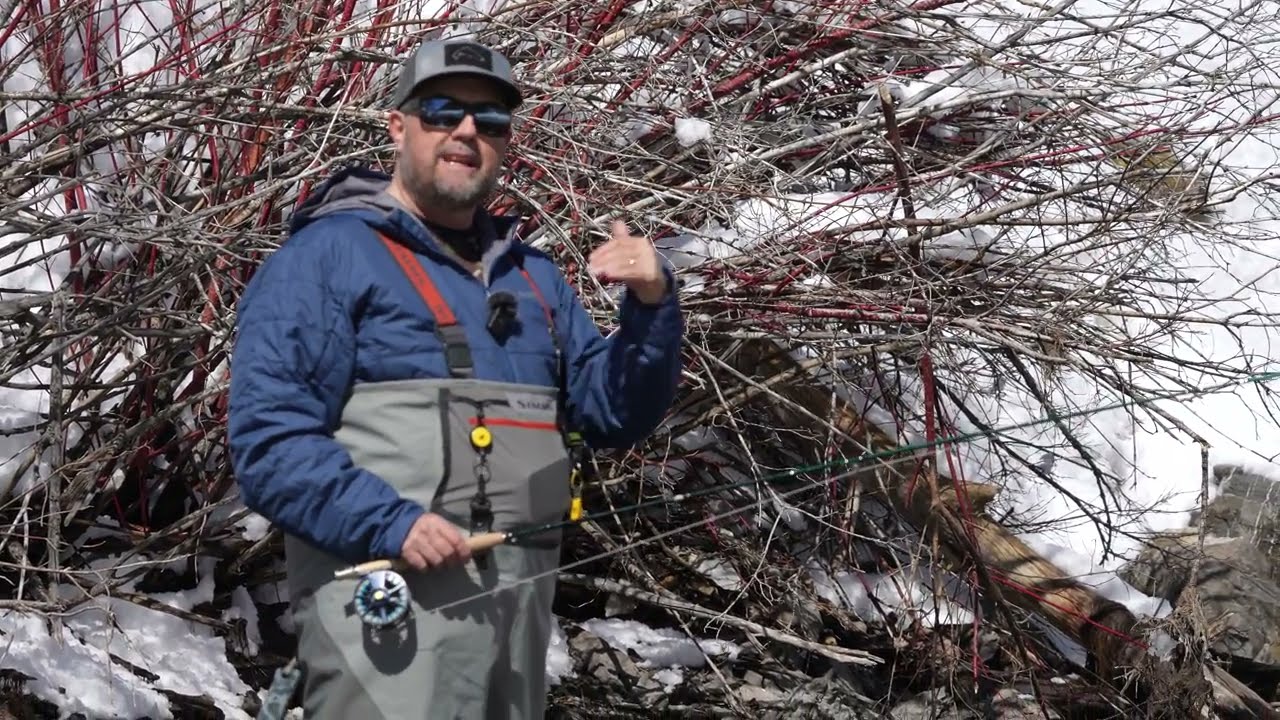The photograph, taken outside in the winter, captures a man standing amidst a snowy landscape. He is dressed in gray fishing overalls with distinctive red suspenders, over which he wears a blue windbreaker. A gray hat and black sunglasses, reflecting the overcast sky, complete his outfit. The man, in mid-conversation, gestures with his left hand, revealing a wedding band, while holding a fishing rod in his right hand, suggesting a fishing excursion, possibly ice fishing. Behind him, the scene features a fallen tree with exposed roots and tangled branches, along with other dead bushes, all partially covered in snow. The sky above is heavily clouded, adding to the wintry atmosphere.